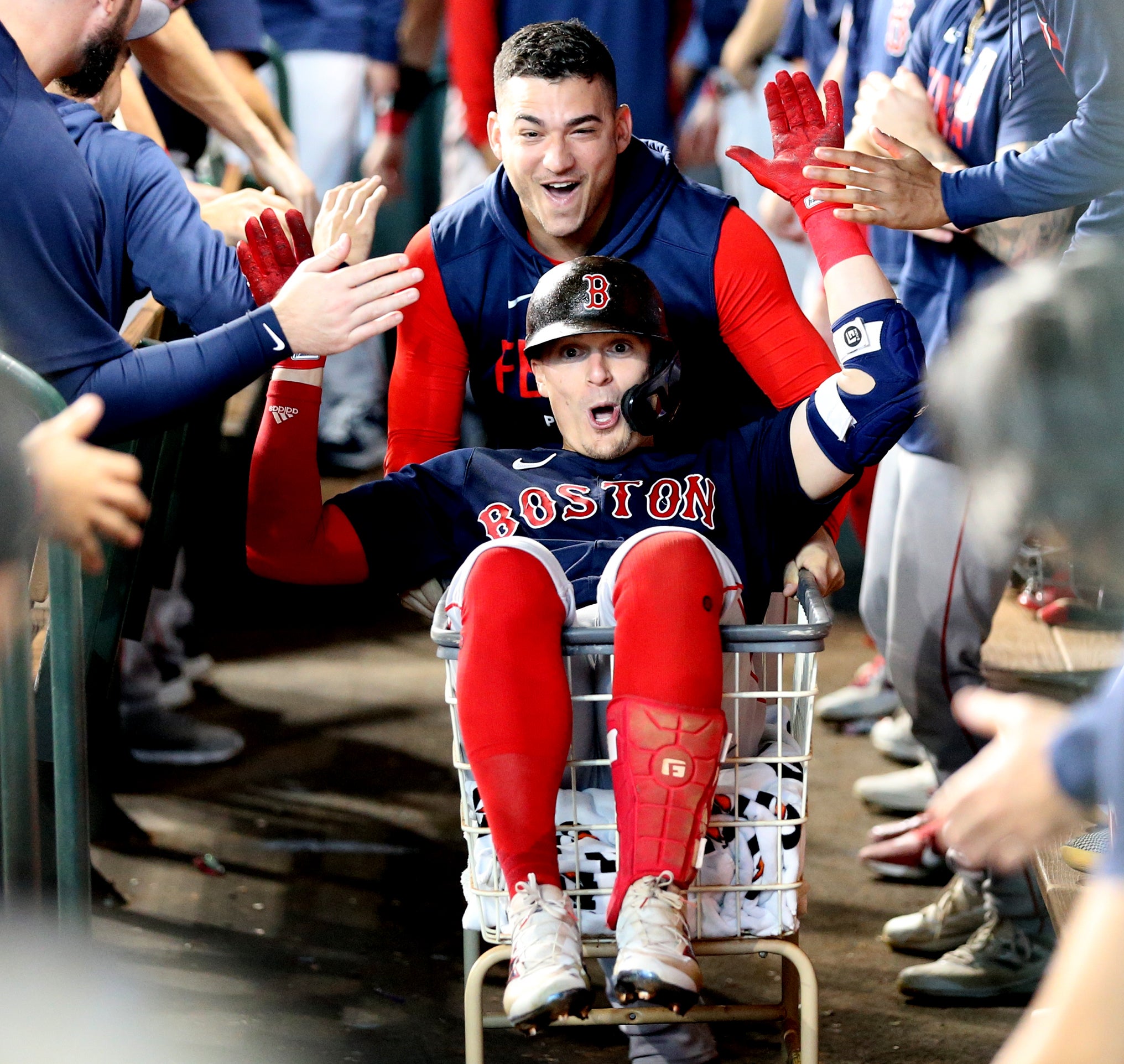In the photo, two Boston Red Sox players are at the center of a joyous scene in the dugout. One player, wearing a typical Boston Red Sox blue jersey with "Boston" emblazoned in red letters, white pants, and full knee-length red stirrups with white cleats, is sitting in a shopping cart's basket as another player pushes him through the dugout. Both players are surrounded by teammates on either side, all celebrating and giving high-fives. The image captures the excitement and camaraderie among the team members who are leaning over a green railing on the left side of the scene. The teammates, dressed in long-sleeved, blue Boston jerseys, some donning red batting gloves, are all part of this lively moment in the dugout, not regular fans in the stands. The overall mood suggests they are celebrating a significant success together.